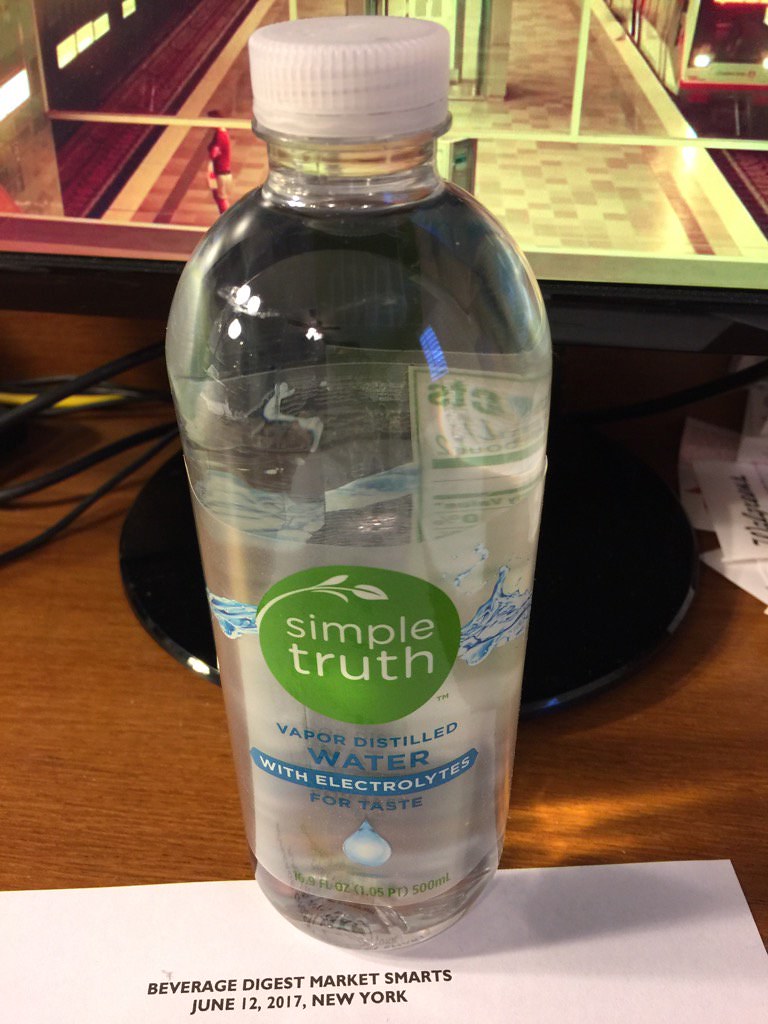The photograph showcases a clear plastic bottle of Simple Truth water, prominently placed on a brown tabletop. The bottle has a white plastic lid and is sealed, indicating it is unopened. The label on the bottle is a green circle featuring the Simple Truth logo, which includes a leaf motif. The label text reads "vapor distilled water with electrolytes for taste" and specifies the volume as "500 milliliters" or "16.9 fluid ounces." The bottle is partially resting on a white piece of paper that bears the text "Beverage Digest, Market Smarts, June 12, 2017, New York." The background reveals a showroom or office setting with brown flooring, a computer screen, visible wires, and some scattered papers to the right-hand side. The bottle's design includes blue swirls around the label, providing a visual contrast to the green and white logo.